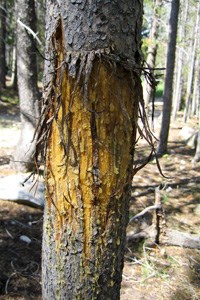In this small, vertical, low-resolution photograph, the foreground is dominated by a tree trunk that appears to have been violently and destructively shredded, exposing a golden-orange wood beneath. The bark is torn off in a jagged, uneven manner, hanging down like fringe, indicating claw-like marks possibly from a large animal. Surrounding the tree trunk, the background features hints of green foliage amidst other tree trunks, with a forest floor scattered with branches, leaves, and debris, suggesting a dense, woodland setting.